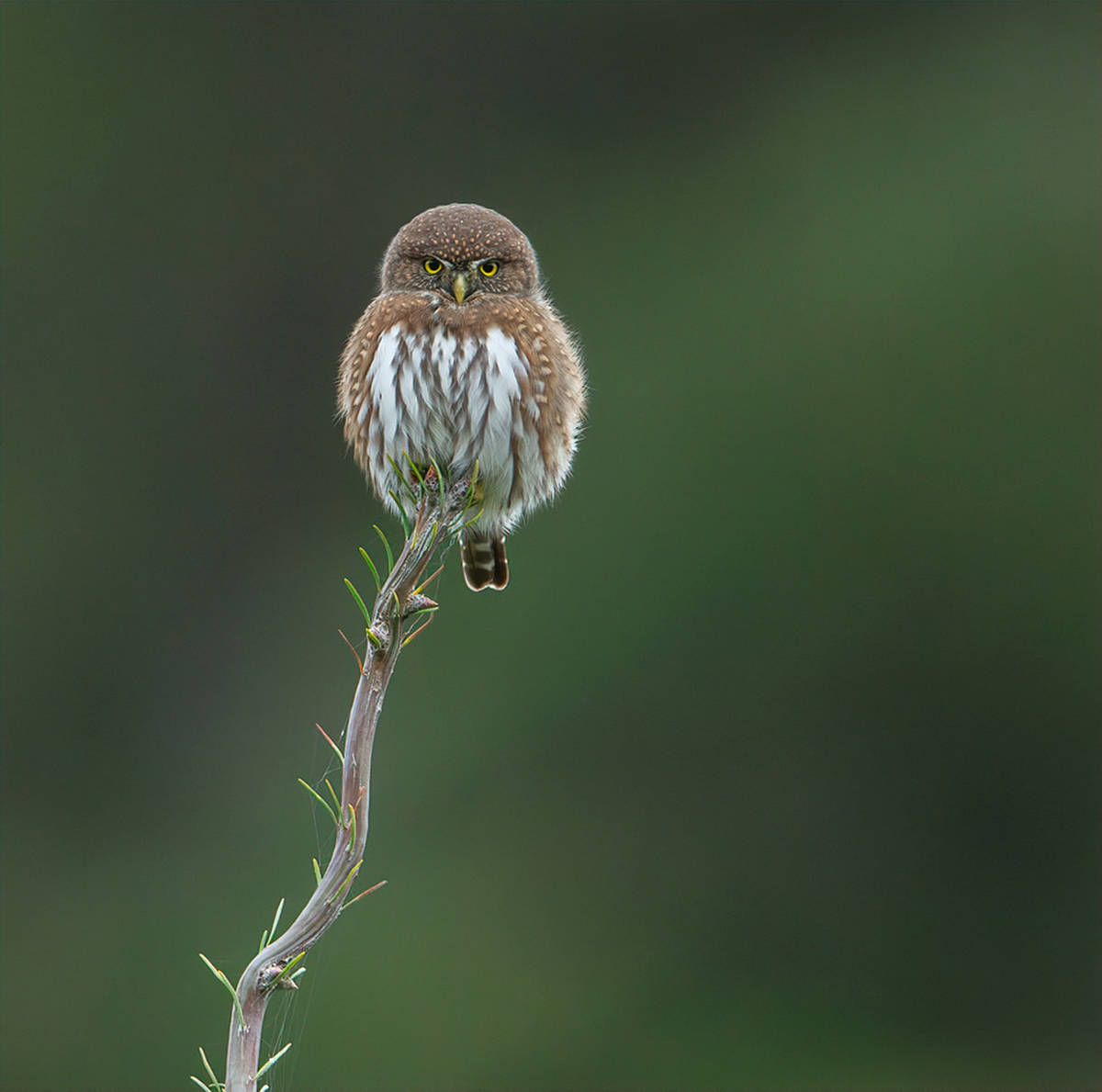This photograph captures a serene moment featuring a northern pygmy owl perched on a slender vertical twig, likely from a pine tree, situated in the bottom left corner of the image. The branch, which is sparsely adorned with green pine needles and a few cobwebs, accentuates the owl's presence. The owl itself is round and fluffed up, resembling an adorable ball or egg. Its head is a soft brown half-circle, adorned with striking yellow eyes and a small golden or orange beak. The owl's body showcases a blend of soft brown and light brown feathers on the wings, transitioning to white and brown on its belly, with distinctive brown and white-striped tail feathers. This endearing creature gazes straight ahead, exuding an aura of alert curiosity. The background is a blurred tapestry of green and blue hues, likely representing out-of-focus trees and foliage, ensuring that the northern pygmy owl remains the central focus of this captivating image.